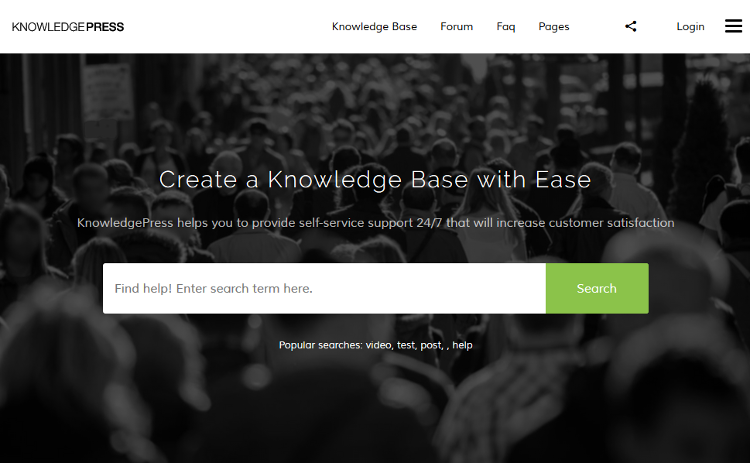A screenshot of the Knowledge Press search screen features prominently. At the very top left corner, "KNOWLEDGE PRESS" is displayed in all caps. The top navigation bar lists the following options from left to right: Knowledge Base, Forum, FAQ, Frequently Asked Questions, Sharing, Icon, Login, and an unexpanded hamburger menu.

Below this, there is a horizontally oriented black and white image, darkened for contrast, depicting a bustling city scene with crowds of people walking both towards and away from the viewer. Superimposed on this image in bold white text are the words, "Create a Knowledge Base with Ease." Beneath this, smaller white text reads, "Knowledge Press helps you provide self-service support 24-7 that will increase customer satisfaction."

Centered below the image is a long white search box with the placeholder text, "Find Help! Enter search term here." To the right of the search box is a lime green button with white text that says "Search."

Below the search box are a series of popular search suggestions listed as: Video, Test, Post, Help. It is worth noting that there is a typographical error after "Post," where two commas are placed erroneously.